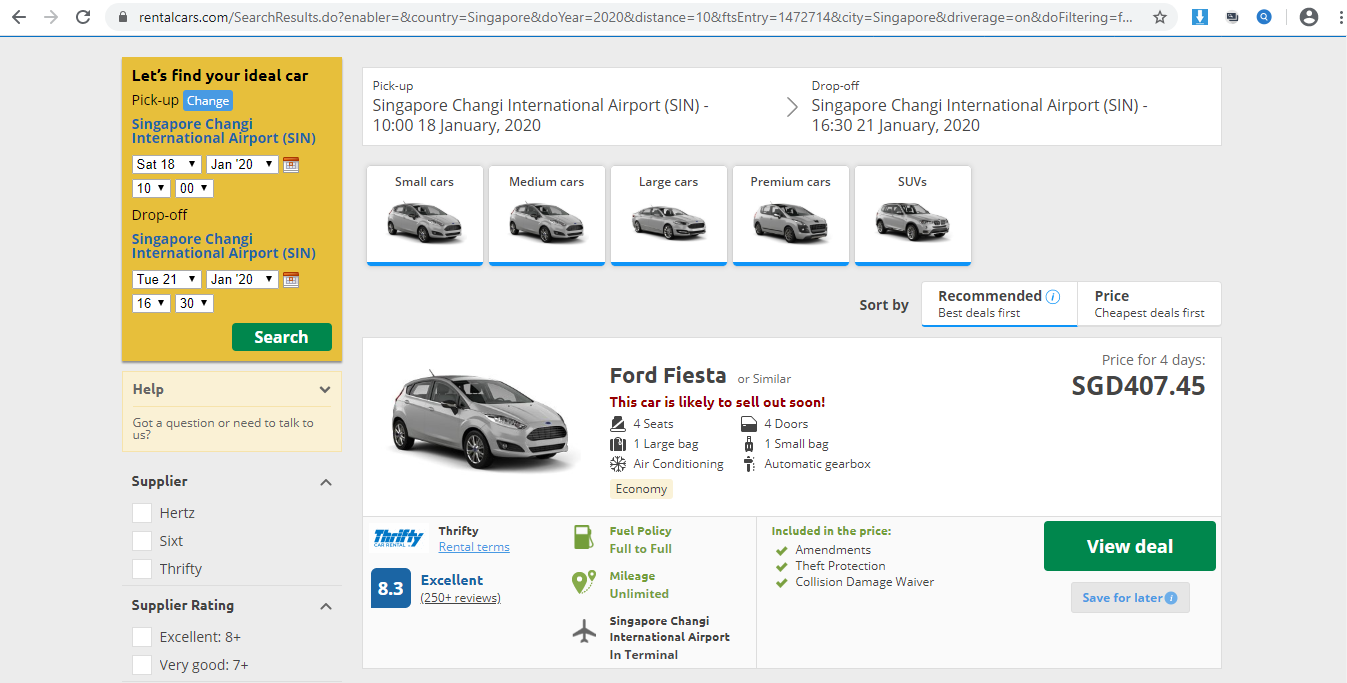This image depicts a rental car booking page on the website RentalCars.com, identifiable by the address bar. The interface includes standard browser navigation icons like left and right arrows, a refresh arrow, and a series of icons to the right, including an unidentified blue icon, another blue icon, a user profile photograph, and three vertical dots for additional options.

On the main section of the page, there's a large yellow box that reads, "Let's find your ideal car." Below it is a form for specifying rental details:
- **Pick-up Location:** Singapore, Singapore - Shanghai International Airport (PVG)
- **Pick-up Date and Time:** Saturday, 18 January 2020 at 10:00 AM
- **Drop-off Location:** Same as pick-up - Shanghai International Airport (PVG)
- **Drop-off Date and Time:** Tuesday, 21 January 2020 at 4:30 PM

Users can adjust these details using drop-down menus and search for available vehicles.

Additional sections include:
- A help section accessible via a drop-down arrow.
- A list of suppliers featuring brands like Hertz and Sixt, along with their ratings (e.g., Excellent 8.8, Very Good 7.0).

The top section allows users to filter vehicles by categories such as Small Cars, Medium Cars, Large Cars, Premium Cars, and SUVs. Sorting options include "Recommended," "Best Deals First," and "Cheapest Deals First."

Highlighted is a featured car — a Ford Fiesta, noted for its likely rapid sell-out. Details of this vehicle include:
- **Capacity:** 4 seats, 1 large bag, 1 small bag
- **Features:** Air conditioning, 4 doors, automatic gearbox
- **Rental Period Cost:** SGD 407.45 for four days
- **Vehicle Type:** Economy
- **Supplier:** Thrifty with an Excellent rating of 8.3
- **Fuel Policy:** Full to Full
- **Mileage:** Unlimited
- **Pick-up/Drop-off:** Singapore, Shanghai International Airport, In Terminal
- **Additional Inclusions:** Price amendments, theft protection, collision damage waiver

Options to "View Deal" or "Save for Later" are available for the user to proceed with their choice.